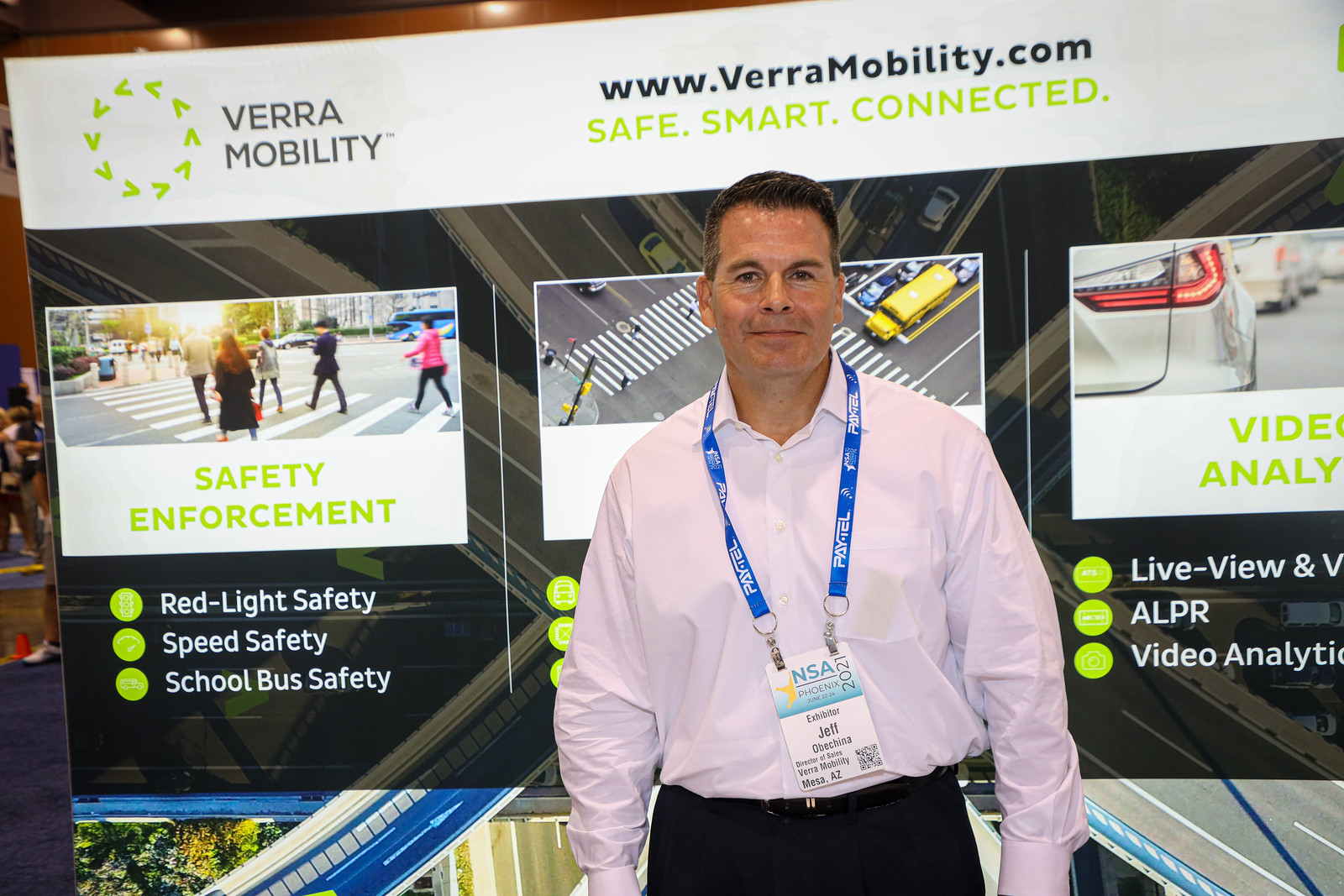This image captures a man standing in front of a large, illuminated sign for Vera Mobility at what appears to be a convention or trade show. He is likely an employee of Vera Mobility and is possibly giving a presentation or managing a booth. The sign prominently features the company's name, "Vera Mobility," with a circular logo composed of arrows at the top left. Above the central portion of the display, the company's website, www.veramobility.com, is showcased, followed by the slogan in green text: "safe.smart.connected."

The man, dressed in a long-sleeved, white, button-down shirt, has short dark hair and is wearing a blue lanyard with the text "NSA" and "2021," along with a name tag at the bottom. The left section of the sign shows a photograph of people walking in a crosswalk with the main features of Vera Mobility listed beneath it: safety enforcement, red light safety, speed safety, and school bus safety. Additional services like video analysis, live view, ALPR, and video analytics are also mentioned, though partially obscured by the man. The right side of the sign includes an image of cars in traffic and another of an intersection with a school bus, emphasizing the company's focus on various safety and analytical services.